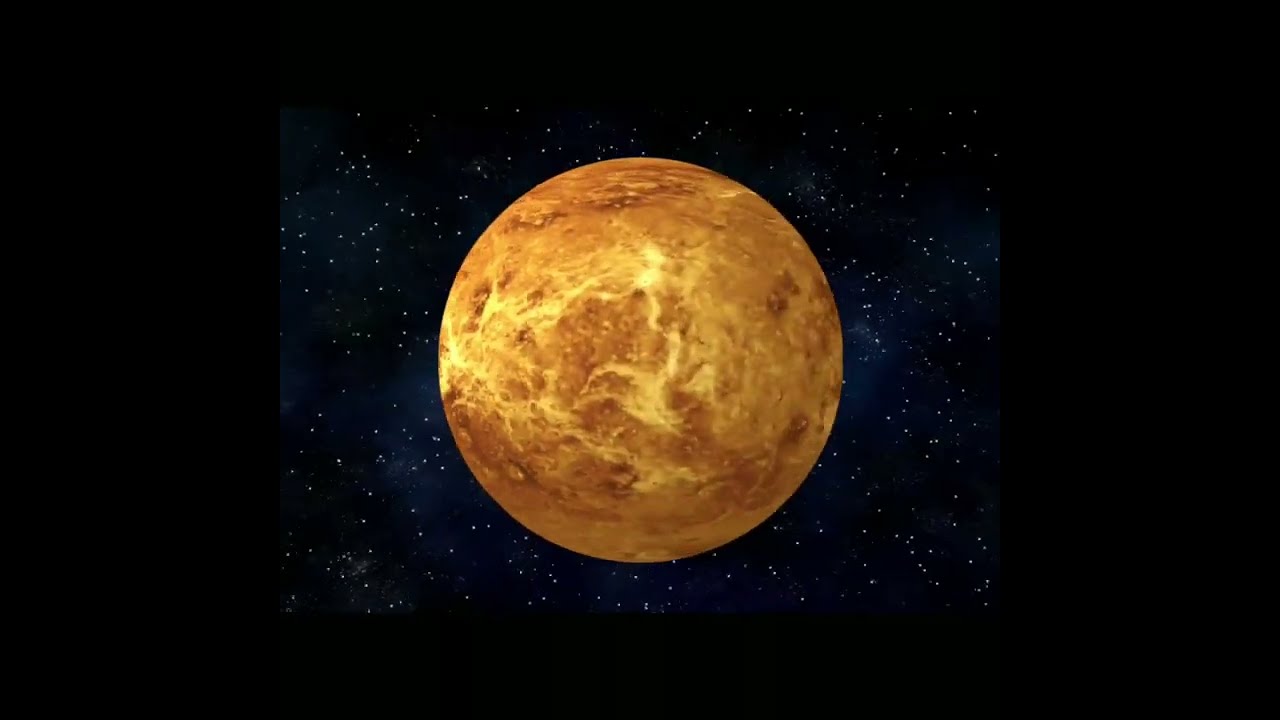In this graphic art image, a large, perfectly spherical planet is prominently displayed in the center of a dark, star-filled space. The planet itself features a blend of orange, yellow, and brown hues, with some areas appearing to glow and others showing white spots that contribute to a blended, textured appearance. Surrounding the planet is a vast expanse of black, characteristic of the deep space backdrop. This dark sky is dotted with hundreds of small, white stars, adding depth and dimension to the scene. The atmosphere around the planet includes regions that are blurry and have a smoky or misty quality, enhancing the overall ethereal and otherworldly ambiance of the image.